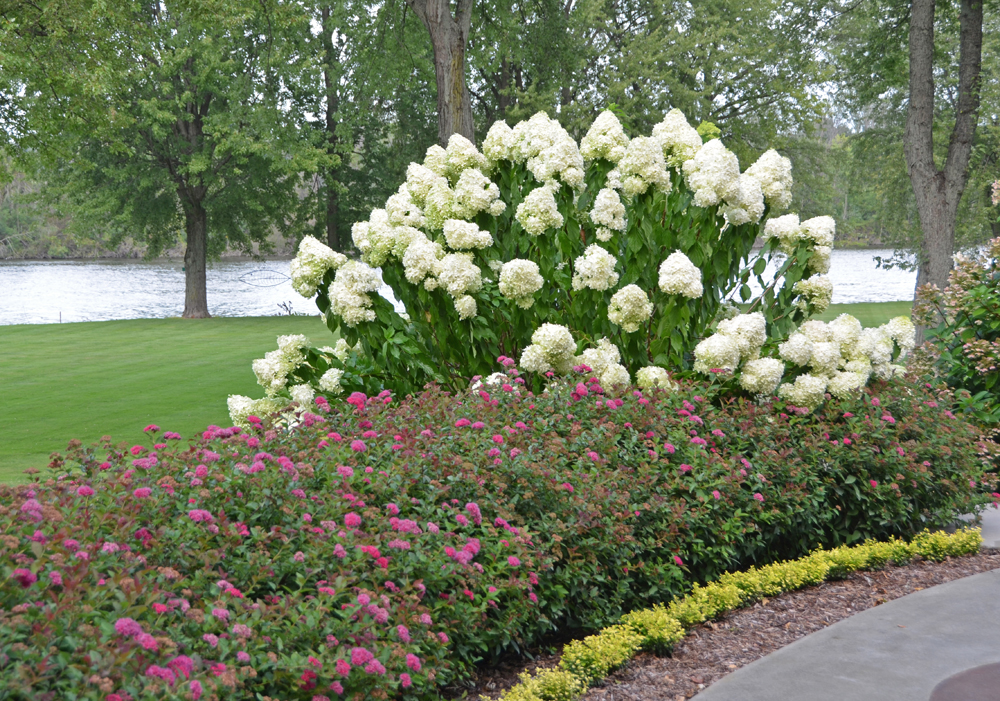This daytime photograph captures a serene outdoor scene in a park-like setting. In the middle of the image, a large plant with bright green leaves and stems blooms with clusters of white flowers, resembling cauliflower. Below and around this central plant, dark green bushes sprout with purple and pink flowers. Directly to the right of this floral arrangement, a forked tree trunk can be seen, with another tree gracing the upper left corner. The background features a well-manicured green grass field stretching towards a calm lake or river, with distant trees lining the horizon under a clear, light blue sky. In the foreground, there's a series of colorful small bushes, including orange-yellow flowers. To the far right of the image, a flat, smooth, gray concrete walking path borders the scene, adding a structured element to this natural landscape.